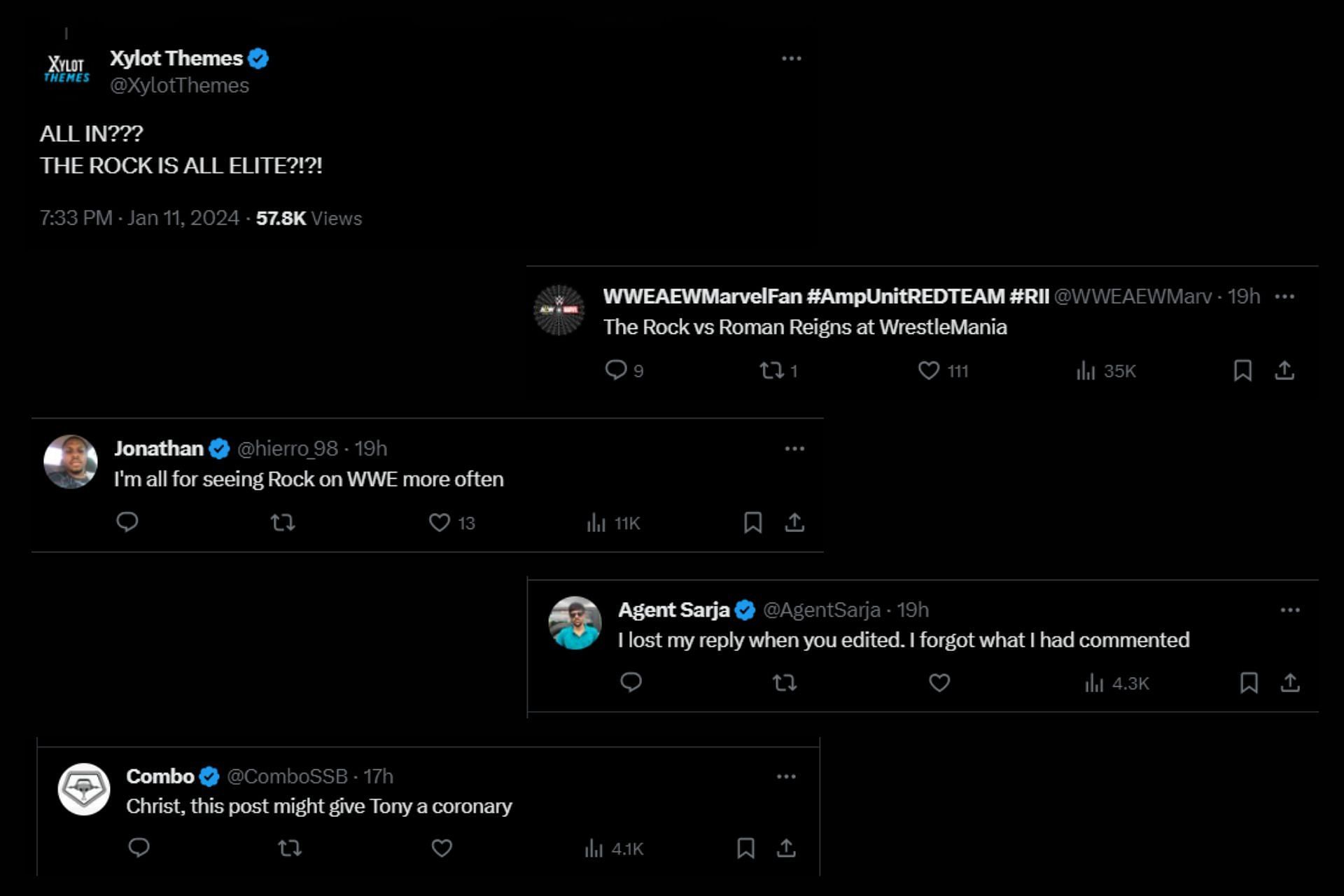This image is a screenshot featuring multiple tweets displayed on a black background. 

At the top, the first tweet is from the user "Xylot Themes" and it reads: "All in??? The Rock is ALL ELITE." This tweet was posted at 7:33 PM on January 11th, 2024, and has garnered 57.8K views.

Below that, to the right, there's a tweet from "WWE AEW Marvel Fan #AMP Unit Red Team #RII" which states: "The Rock vs Roman Reigns at WrestleMania." This tweet has received nine comments, one retweet, 111 likes, and has been viewed 35,000 times.

To the left of that tweet, there is another tweet from a user named "Jonathan" saying: "I'm all for seeing The Rock on WWE more often." This tweet has no comments or retweets, but has 13 likes and 11,000 views.

Beneath Jonathan's tweet, there is a tweet from "Agent Sarah" which says: "I lost my reply when you edited what I forgot what I had commented." This tweet has zero comments, zero retweets, zero likes, and 4.3K views.

Finally, at the bottom left, the last tweet is from "Combo Combo SSB" posted 17 hours ago. It reads: "Christ, this post might give Tony a coronary." This tweet has zero comments, zero retweets, zero likes, and 4.1K views.